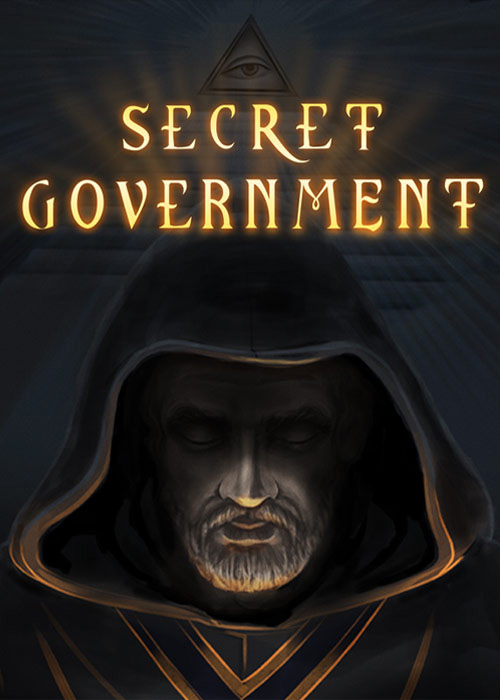The captivating image features a digitally created illustration centered around a hooded man positioned towards the bottom of the composition. The man, who appears to be older with a short beard and dark facial features, is dressed in a black robe adorned with gold accents around the hood and forming a V pattern at the front. His eyes are closed and his expression is solemn.

Above the man, glowing in bright gold lettering, is the phrase "Secret Government," set against a stark black background that makes the text stand out vividly. At the top of the image, there is a prominent triangle with an open eye at its center, resembling a symbolic all-seeing eye, which replaces the usual pyramid imagery. Emanating from the top of the hood are streams of light, adding to the dramatic and mysterious aura of the artwork. The blend of colors—including shades of black, gray, yellow, orange, and silver—contribute to the high-quality, visually striking nature of the piece, suggesting it might be shared on social media or used as conceptual artwork.